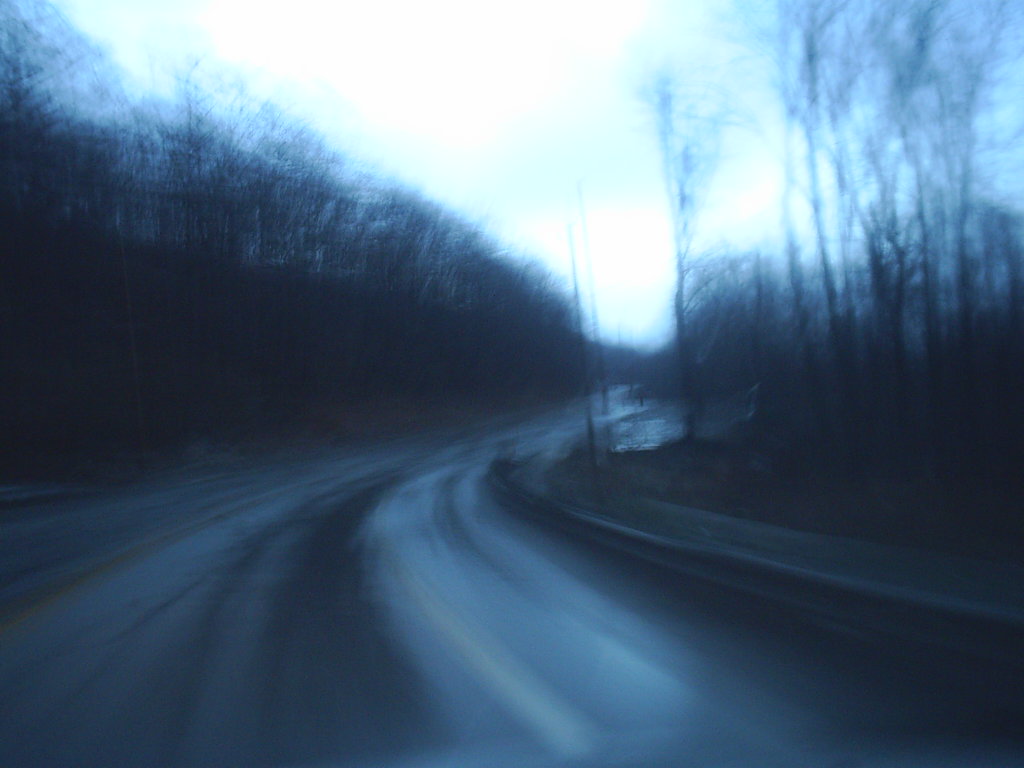This image captures a dark, winding, two-lane highway that starts at the bottom-center and curves towards the back of the scene. The road surface has a sheen, hinting it might have rained recently. There is a yellow line faintly visible on the black asphalt, with a slight bluish hue throughout the image, giving it an almost painterly effect. The sky is a bright yet grayish-blue, suggesting either twilight or moonlight illuminating the scene. Tall, leafless trees line both sides of the road, their scraggly, bare branches accentuating the desolate and possibly wintery atmosphere. To the right of the road is a small sidewalk area, slightly elevated above the dirt and tree line. In the background, the faint silhouette of snow-capped mountains can be discerned through the blur, adding to the ethereal quality of the image. The overall desolate landscape is devoid of cars, underlining its tranquility and solitude.